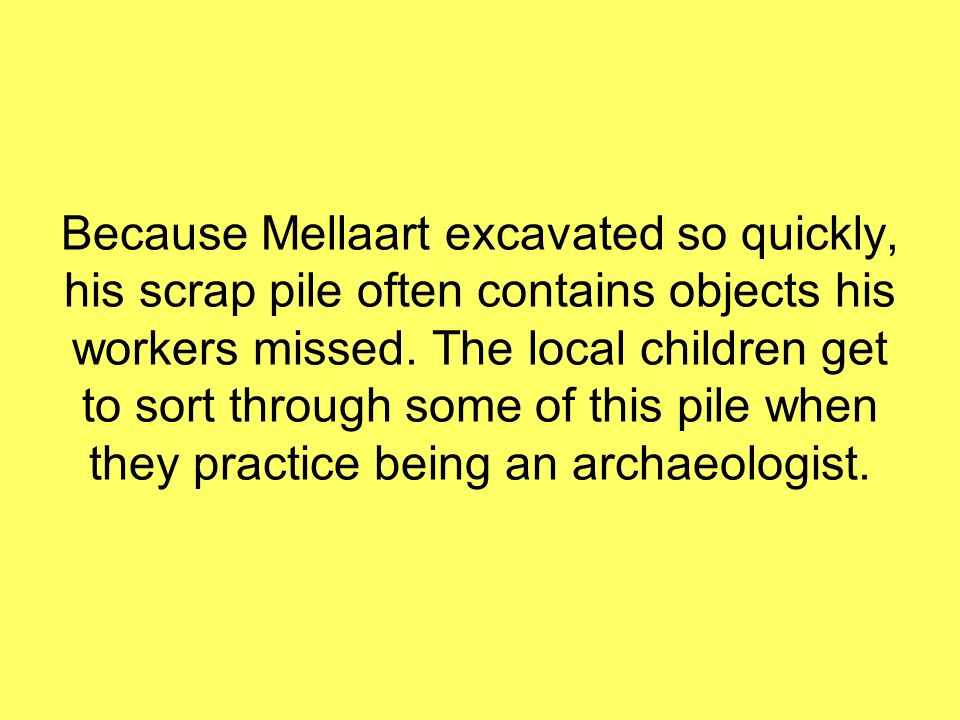The image depicts a plain, bright canary yellow background with a centered paragraph of black text. The text is easy to read, written in a fairly large Arial font. It states, "Because Mellart excavated so quickly, his scrap pile often contains objects his workers missed. The local children get to sort through some of this pile when they practice being an archaeologist." The text is arranged in five lines without any indentation, creating a high contrast and eye-catching visual.